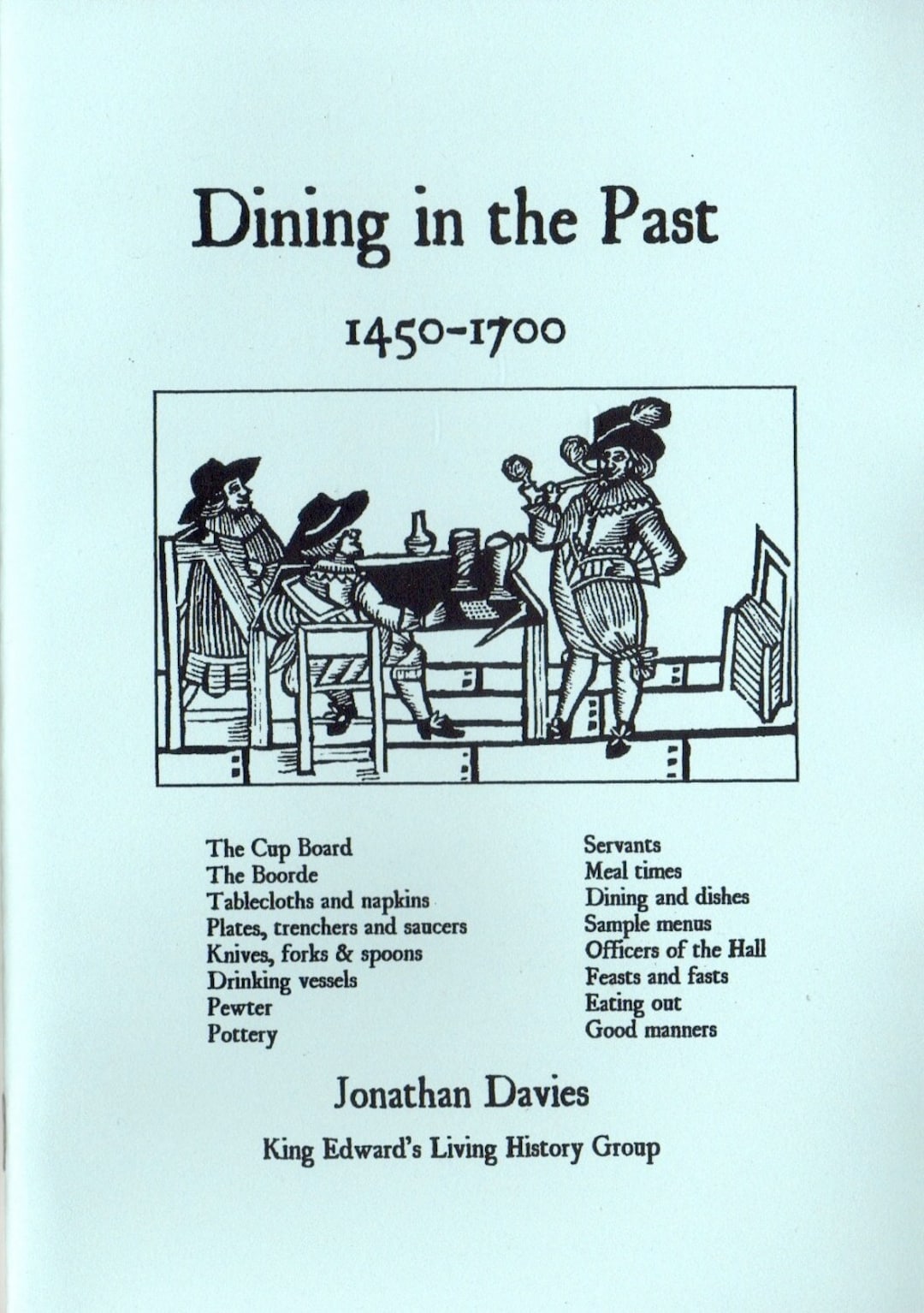The image depicts a rectangular, light blue cover of a book titled "Dining in the Past: 1450 to 1700," written in black text at the top center. Directly below the title and date is a black rectangular illustration showing three men in historical attire from the 1600s, two of whom are sitting at a table and one standing to the right, smoking a pipe. They are depicted on a wooden plank floor. The cover also features two columns of text listing various historical dining topics such as "the cupboard, the board, tablecloths and napkins, plates, trenches and saucers, knives, forks and spoons, drinking vessels, pewter, pottery" on the left, and "servants, mealtimes, dining and dishes, sample menus, offices of the hall, feasts and fasts, eating out, good manners" on the right. The author, Jonathan Davies from King Edward's Living History Group, is noted at the bottom.